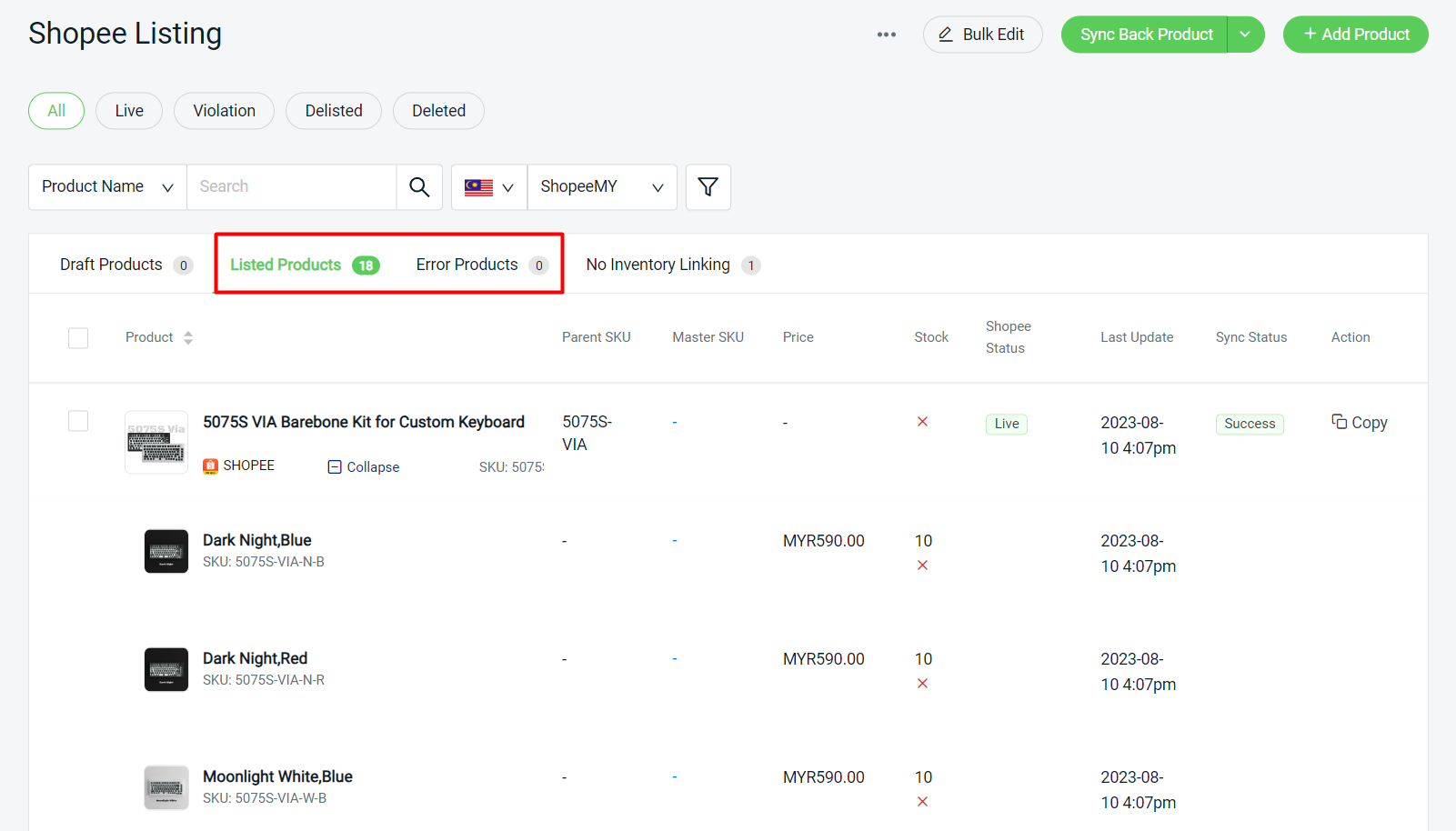The image displays a partially visible, horizontally-oriented rectangular interface, with its lower portion cut off. The interface appears to be an educational screenshot or demo related to managing product listings on the Shopee platform.

In the upper left corner, the label "Shopee Listing" is prominently featured in black text. On the upper right side of the interface, there are several controls:
- Three vertically arranged dots.
- A grey button labeled "Bulk Editor" with a pencil icon.
- A light grey button with a darker grey outline and black text labeled "Sync Back Product," accompanied by a downward arrow indicating a dropdown menu.
- A green button with white text labeled "Add Product" with a plus sign.

Below the "Shopee Listing" label, there is a set of navigation buttons, each available for different listing statuses:
- "All" (highlighted in white with a green font and outline)
- "Live"
- "Violation"
- "Delisted"
- "Deselect"
- "Deleted"

These buttons are grey with black text, except for the active "All" button.

Further down, the interface contains a series of product names, associated with a dropdown search bar labeled "Search." There are additional dropdown options labeled "American Flag" and "My Shopee."

Moreover, the interface provides a summary of product statuses:
- "Draft Products: 0"
- "Listed Products: 18"
- "Error Products: 0"

The "Error Products" section is highlighted with a red rectangle around the corresponding text.

Overall, the interface layout and elements suggest it is intended for instructional or educational use, guiding users on how to navigate and manage product listings within the Shopee platform.